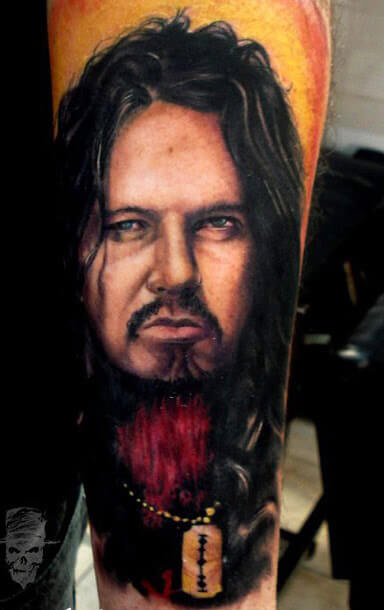This detailed close-up photograph captures an intricately designed tattoo on a person's arm. The tattoo is a vivid portrait of a steely-eyed man who exudes a rock star demeanor. He has long, wavy, brownish-black hair cascading around his face and sports dark eyebrows, eye bags, and a distinctive facial hair combination of a dark mustache and goatee, both of which frame his pronounced pout. His light blue eyes stand out, staring intensely straight ahead. The man's expression conveys a mix of anger and determination. Around his neck, he wears a gold chain with a pendant that resembles a razor blade. His attire is somewhat ambiguous but includes black and red elements around the chest and neck area. Additionally, in the tattoo's bottom left corner, there is a small image of a skull, which could be interpreted as a logo. The level of detail in the tattoo is quite impressive, making it a remarkable piece of body art.